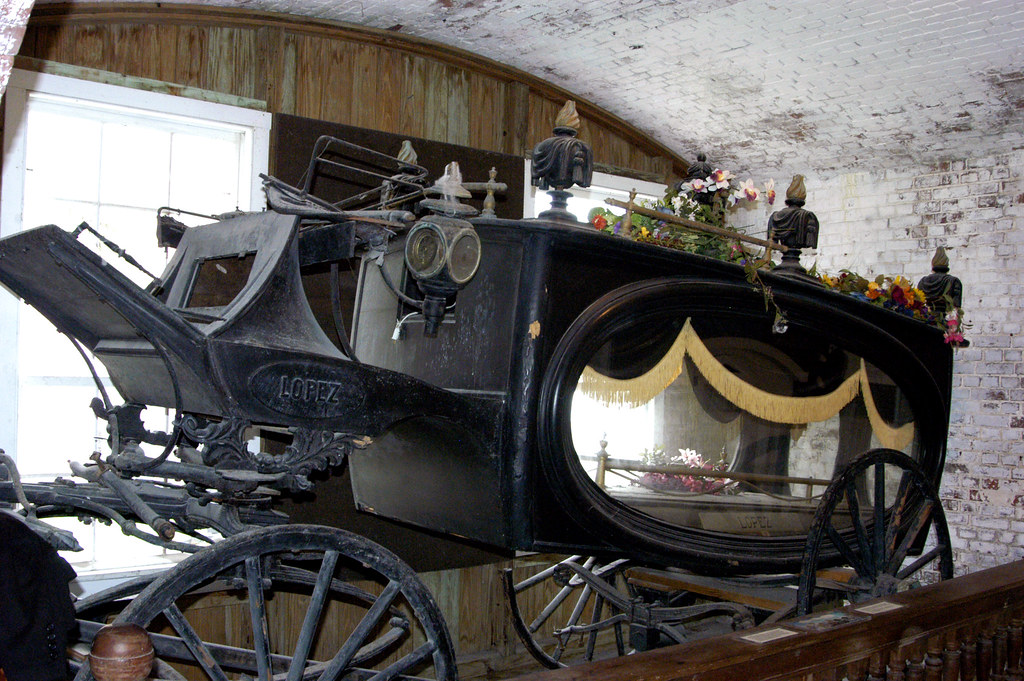This indoor daylight color photograph captures an antique black hearse wagon, suggesting it is part of a museum display located in a small room with a curved, whitewashed brick ceiling and walls, complemented by a brown wooden end wall adorned with large windows. The hearse, notably large and entirely black, features a driver's seat at the front with a black hooded lantern beside it. Decorative rails with flourishes on the corners run along the top, where a display of flowers hints at how it might have been used historically. The hearse stands on large wooden wheels and showcases an oval side window adorned with velvet drapes fringed around it, providing a view of the casket platform within. Bronze-like bars are present to secure the casket, and a flower arrangement on the platform further illustrates its original purpose. A sign on the side reads "Lopez," possibly indicating the brand. Visitors are separated from the hearse by a wooden rail, with small signs or placards likely detailing the history and provenance of the exhibit.